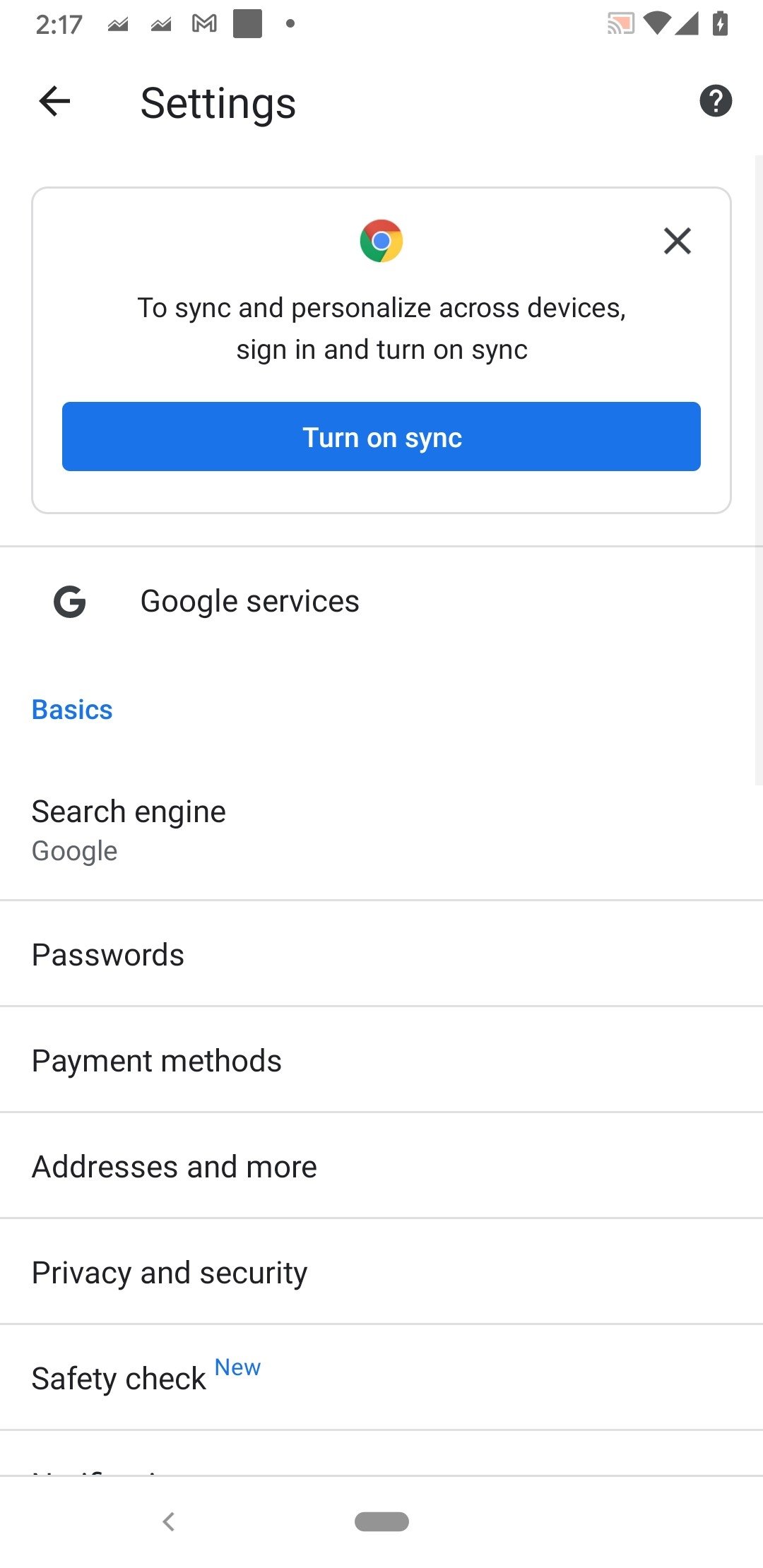The image showcases a smartphone screen displaying the settings menu for Google Chrome. The background is white. In the top left corner, the time is shown as 2:17 PM in dark gray font. Adjacent to the time, there are two signal indicators: one appears to represent mobile signal with gray bars, and the other symbolizes a gray and white bar chart. Next to these indicators is a white 'M' outlined in gray, likely representing the Gmail app. There is also a gray square icon with a small gray circle within it. On the top right, the fully gray Wi-Fi icon, signal reception symbol, and battery indicator (which has a white lightning bolt in it) are visible.

Below these icons, on the left side, there's a black arrow pointing to the left, indicating a back function. Next to it, the word "Settings" appears in black text. Nearby, there's a black circle housing a white question mark. Moving downwards, a gray rectangle encompasses the Google Chrome logo and black text that reads, "To search and personalize across devices, turn on sync." Beside this text, in a blue rectangle with white font, is the prompt, "Turn on sync."

A thin gray line spans across the screen, segmenting the interface. Below this line, in black text, is "Google services." Beneath that, the word "Basics" appears in blue. The subsequent sections, each separated by thin gray lines, include options in black text: "Search engine Google," "Password," "Payment method," "Addresses and more," and "Privacy and security." At the bottom, the section labeled "Safety check" has the word "new" highlighted in blue in the corner.